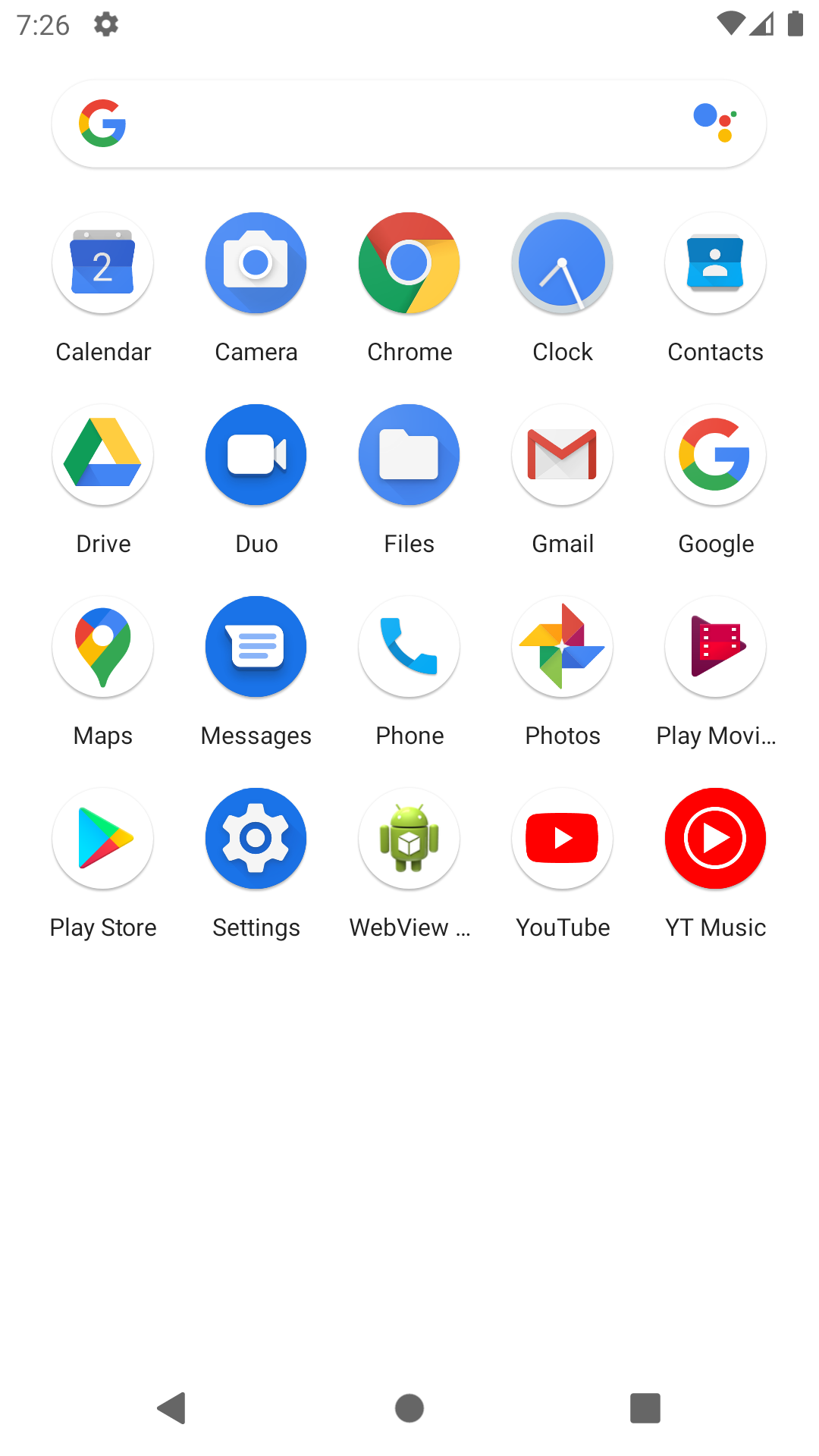This is a detailed screenshot captured from a cell phone, displaying the home screen interface. At the top center of the screen, the time "7:26" is prominently shown. To the left of the clock is a gear icon, indicating the settings option. Below the time and gear icon, the Google search bar is placed, adorned with the multicolored 'G' logo, consisting of a large blue circle, next to smaller red and yellow circles. 

Directly below the search bar is an array of application icons, likely situated in the settings section of the phone. The icons are displayed in a grid pattern and include:

- Calendar
- Camera
- Chrome
- Clock
- Contacts
- Drive
- Duo (resembles a FaceTime icon)
- Files
- Gmail
- Google
- Maps (marked with a location pin)
- Messages
- Phone
- Photos
- Play Movies
- Play Store
- Settings
- Web View
- YouTube
- YouTube Music

At the very bottom of the screen, there's a solid gray circle, flanked by a solid gray left arrow on the left, and a solid gray square on the right.